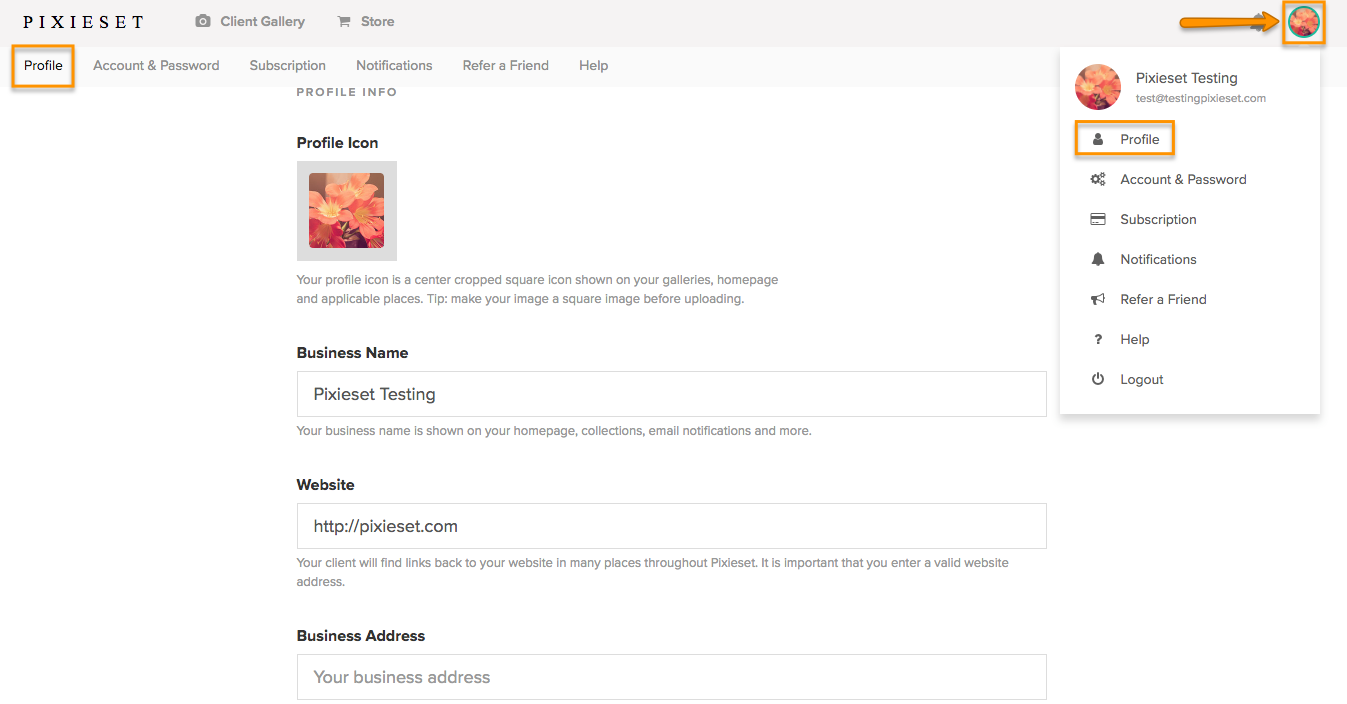The image displays the profile screen of a platform called Pixie Set. On this screen, users have the option to update their profile icon, which is noted to be a center-cropped square image visible on the gallery's homepage and various application interfaces. It is recommended that users ensure their image is square before uploading.

Additionally, users can input their business name, associated website, and business address if applicable. On the right side of the screen, there is a dropdown menu accessible from the designated profile icon. This menu displays the business name and offers several options, including a route back to the current profile screen and various other features such as account settings, password changes, subscription details, notifications, referral opportunities, help resources, and a log-out option.

The same options found in the dropdown menu are also available in a more traditional menu layout along the top of the screen, running from left to right, starting with the profile section.